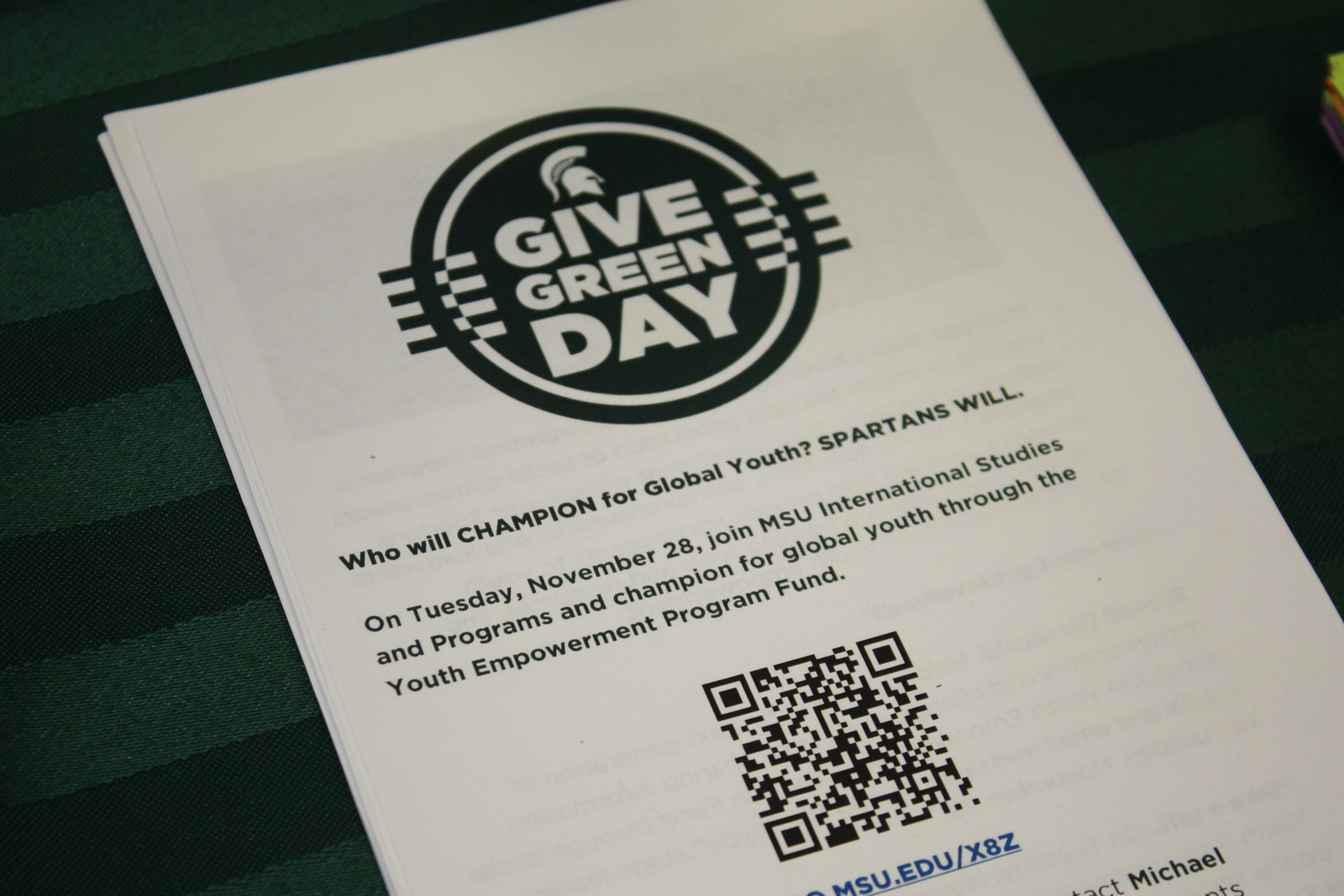The image showcases a single page from a folded white pamphlet or program, laid out on a green striped fabric that appears to be a tablecloth. At the top of the page, there is a dark green circle featuring a white Spartan helmet emblem, above the bold white text "Give Green Day." Below this logo, black text reads, "Who Will Champion for Global Youth? Spartans Will." Further down, an announcement states, "On Tuesday, November 28th, join MSU International Studies and Programs and champion for global youth through the Youth Empowerment Program Fund." Central to the lower part of the page is a QR code, with a blue URL displayed beneath it.